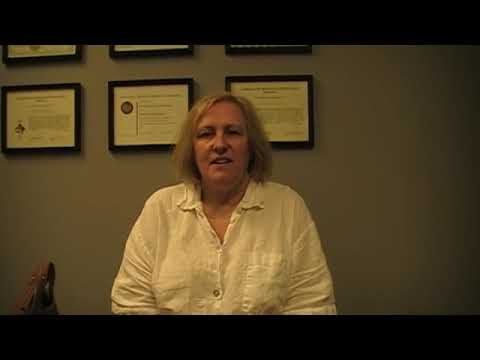The image depicts a middle-aged woman with short, almost shoulder-length blonde hair, sitting indoors in front of a grayish-beige wall adorned with six framed certificates or awards. She is wearing a white button-down long-sleeve shirt and appears to be speaking to the camera, with a slight smile and her mouth slightly open. The frames behind her are arranged in two rows of three, with the top row partially cropped out of the image. The scene suggests she might be a professional, possibly a teacher, business leader, principal, or dean. To her left, partially visible, is an object that could be a bag or pencil holder, adding a personal or professional context to the setting. The photograph has a slightly lower quality, characteristic of an older camera, and features black bars across the top and bottom.